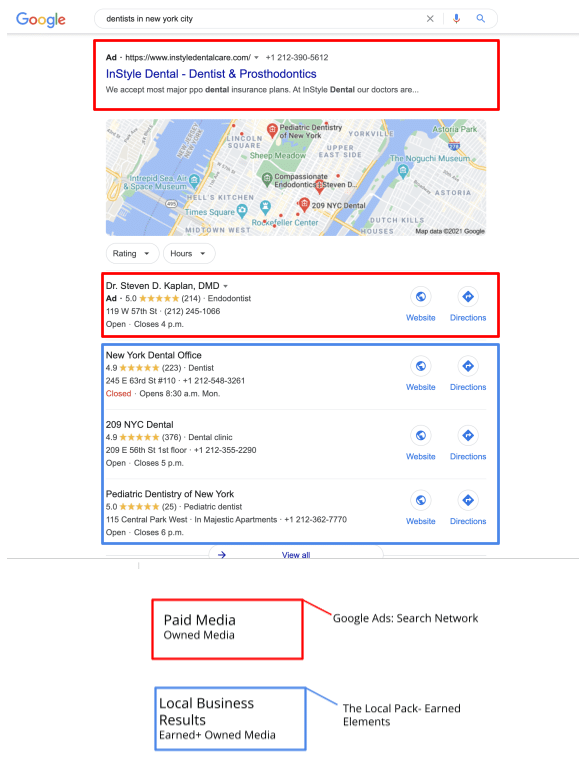Here is the cleaned-up and detailed caption:

---

The screenshot captures a portion of a Google search results page. At the top, the search bar contains the query "dentist in New York City." Despite being zoomed in, the text remains quite small and challenging to read. Immediately below the search bar, there is a paid advertisement for "InStyle Dental - Dentists and Prosthodontics," which notes it accepts the most major PPO dental insurance plans.

Following the advertisement, a section displays a Google Maps image of Manhattan, highlighting neighborhoods such as Harlem and the East River, along with parts of New Jersey and Queens.

Beneath the map image, a red-outlined box provides details on Dr. Steven D. Kaplan, DMD, an endodontist with a 5.0-star rating based on 214 reviews. His practice is located at 119 West 57th Street, and the phone number begins with 212-245 (the remaining digits are unclear). The listing mentions that the office closes at 4 p.m.

A second box, outlined in blue, includes information about "New York Dental Office," followed by a mention of "209 NYC Dental."